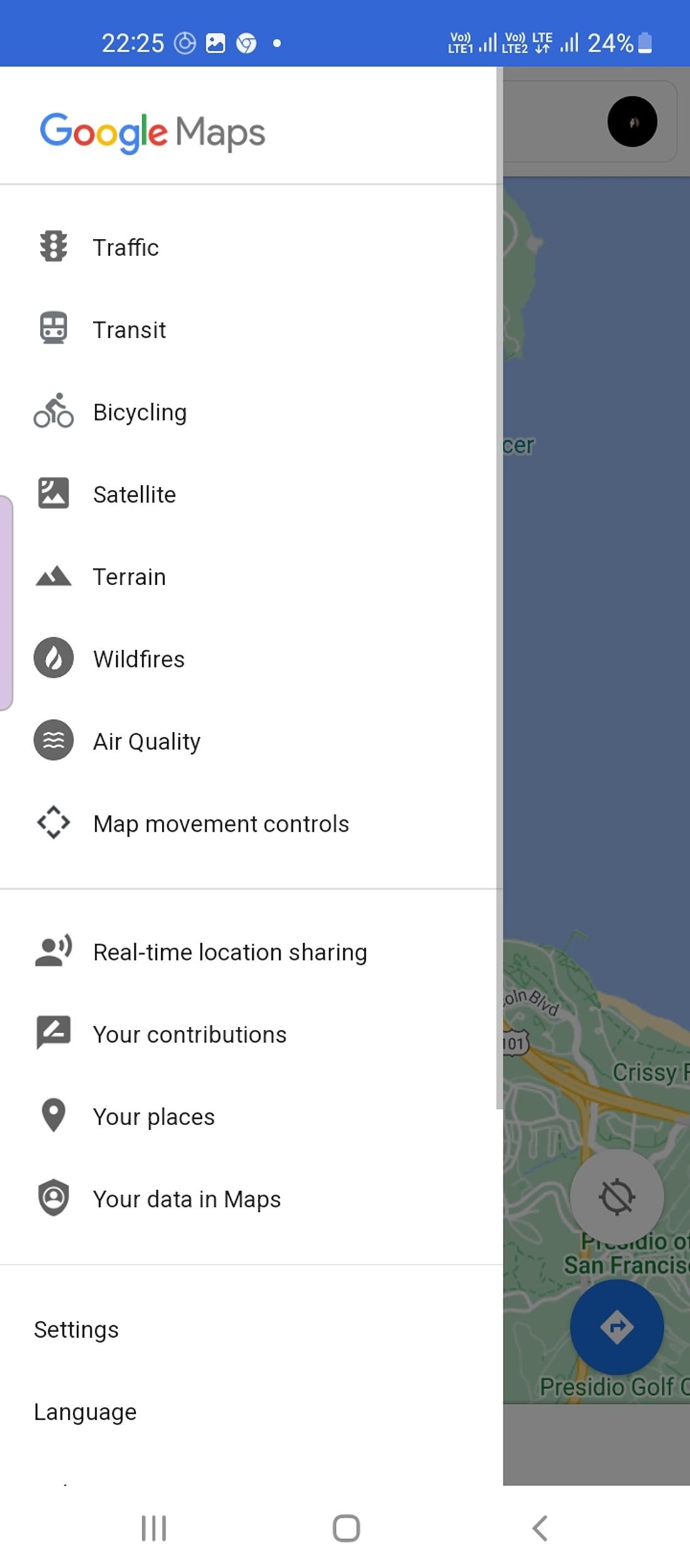A detailed screenshot of a Google Maps page on a mobile device. The majority of the screen is occupied by a white pop-up window with "Google Maps" prominently displayed at the top, underlined by a dividing line. Below the title, the interface is segmented into two main sections, featuring vertical rows of buttons with icons to the left and descriptive text to the right.

The first section includes options for various map views and functionalities like Traffic, Transit, Bicycling, Satellite, Terrain, Wildfires, Air Quality, and Map Movement Controls. Each of these options is aligned vertically and separated by a horizontal line.

The second section contains personalized and interactive features such as Real-time Sharing, Your Contributions, Your Places, and Your Data in Maps. This is followed by another dividing line, after which Settings and Language options are listed.

To the right of the pop-up window, a small portion of the actual map is visible, depicting what appears to be a body of water. At the very bottom of the screen, two prominent buttons are located: a rectangular button with a strikethrough and a blue button labeled "Directions."